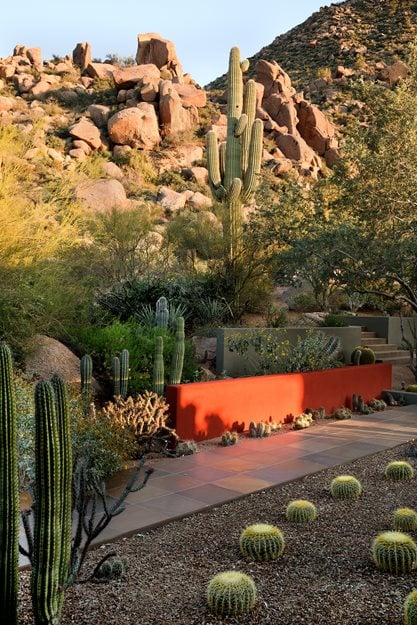The image depicts a meticulously arranged desert garden set against a backdrop of orange-hued hills and rocky formations. At the top of the image, a clear, light blue sky stretches above. The centerpiece of the garden is a towering green saguaro cactus flanked by lush green bushes. Below it, several long, spiky cacti cluster near the left-hand side. The garden features an orange half-wall and a small flight of stairs near the right-hand side, leading up to the prominent cactus. Sprawled across the gravelly soil at the bottom are numerous spherical cacti. A sidewalk cuts through the scene, lined to the left by young cacti and various desert plants, accentuating the man-made elements amidst the natural beauty. The sun casts shadows across the landscape, highlighting the vibrant colors and textures of this desert oasis.